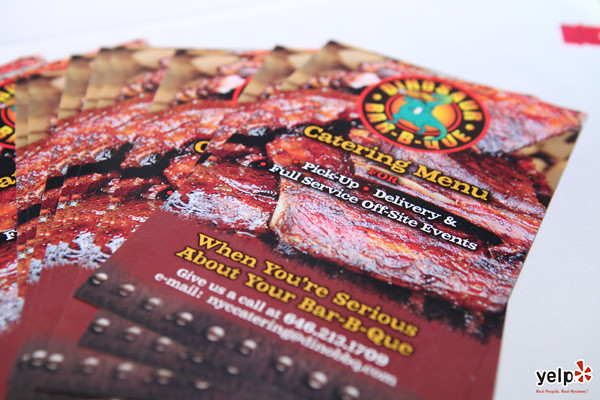This image displays a stack of vibrant, red-themed catering menus for a barbecue restaurant, scattered haphazardly across a white surface, potentially a table. Dominating the layout, a central brochure presents an enticing close-up of barbecued ribs, overlaid with essential details. The upper portion of the menu features a logo comprising a red circle encasing a blue dinosaur, marked as "Bingham's Barbecue" in circular fashion, bordered in red. Below this, bold yellow text announces "Catering Menu," accompanied by white text offering services for pickup, delivery, and full-service off-site events. The lower half emphasizes the slogan "When you're serious about your barbecue" in yellow print against a darker red background, supplemented with a contact number and email. The bottom right corner of the image subtly includes the black Yelp logo with a red star, suggesting a potential advertisement for Yelp. The slightly askew arrangement of the brochures, combined with the photographer’s angled perspective, adds a casual, dynamic flair to the image.